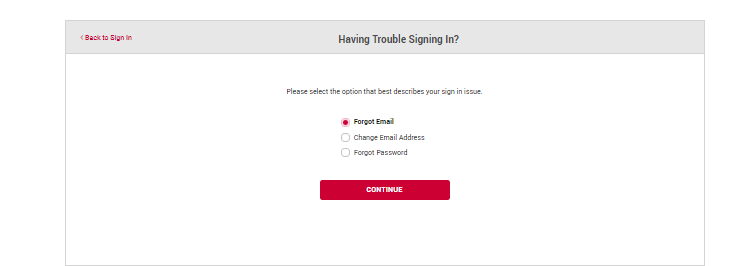The image depicts a webpage designed to assist users experiencing issues with signing in. The top section features a gray banner that includes a red "Back to Sign In" button accompanied by a back arrow. Dominating the page is a prominent header that reads, "Having trouble signing in?" followed by a prompt: "Please select the option that best describes your sign-in issue."

Below this prompt, there are several selectable options:
1. Forgot email
2. Change email address
3. Forgot password

The selected option is highlighted in bold black, indicating "Forgot email" as the current choice. When an option is selected, it turns red and the text is bolded for emphasis. At the bottom of the options list, there is a prominent red "Continue" button with white lettering. The overall design is simple and user-friendly, providing a clear path for users to resolve their sign-in issues efficiently.